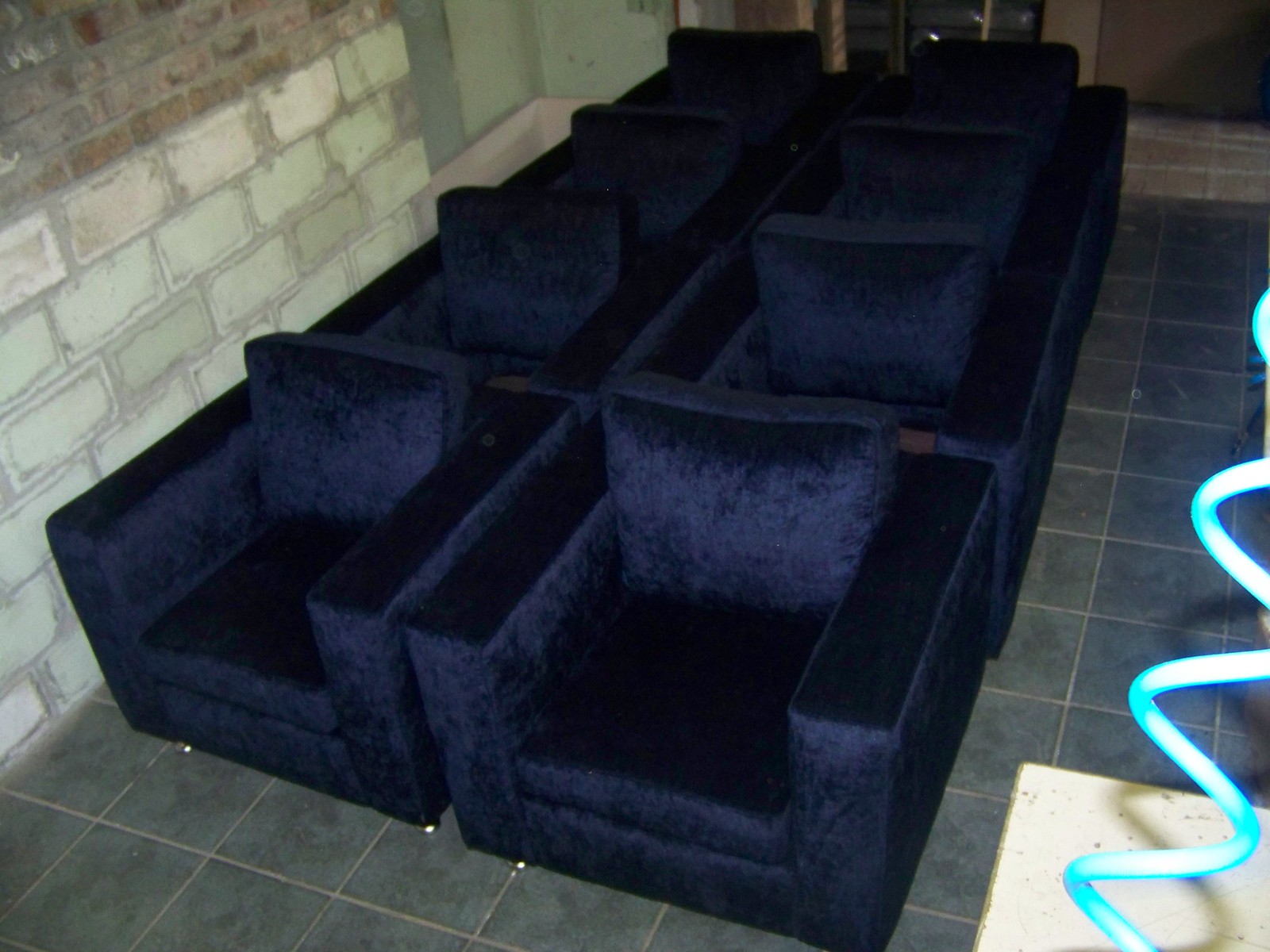This is a color photograph taken indoors from an overhead perspective, capturing a set of eight plush, dark blue velvet armchairs. The chairs are arranged in four rows of two, positioned side by side and facing slightly towards the bottom right corner of the frame. They rest on dark grey square tiles. Each chair features a square design with two cushions—one for seating and one for back support.

A white brick wall runs along the left side of the image, transitioning to smaller greyish bricks towards the top. In the background, there is also a hint of a glass door or window. A ledge is visible at the top of the photograph, behind the chairs. At the bottom right corner, a white square stand is present, accompanied by a blue cable that spirals upward towards the middle of the picture, somewhat washed out by the camera flash. The tiny feet of the front chairs can be seen peeking from underneath them, adding to the intricate detailing of the layout.